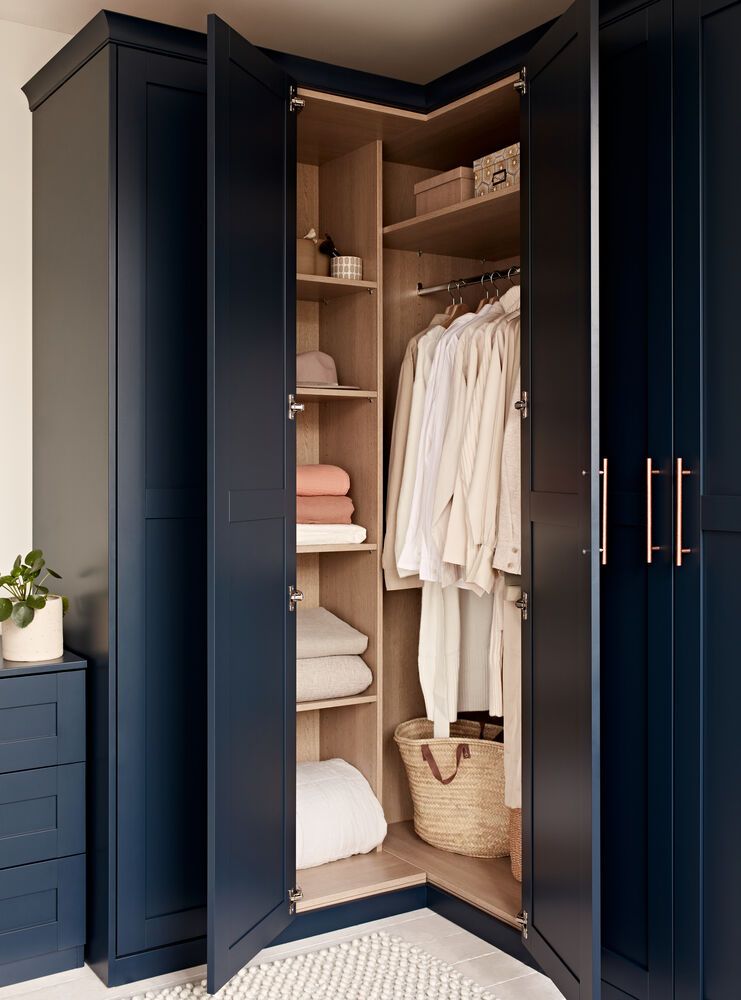The image depicts a modern, tall, navy-blue cabinet standing against a white wall and floor. Unlike a built-in closet, this cabinet appears as a piece of furniture with a satin-like finish and gold hardware, showcasing sleek and contemporary design. The cabinet doors are open, revealing a well-organized interior. Inside, several natural brown wooden shelves hold folded towels in white and pink hues, alongside baskets and boxes, likely containing toiletries. On the right side of the cabinet, a bar is fitted with numerous hangers organizing white garments, including robes and possibly a few shirts. Below these hanging clothes sits a fabric basket with indeterminable contents. Adjacent to the cabinet, there is a small table matching the cabinet's navy color, topped with a potted plant in a white pot. The setting is completed by a section of tiled floor extending to a rug nearby.